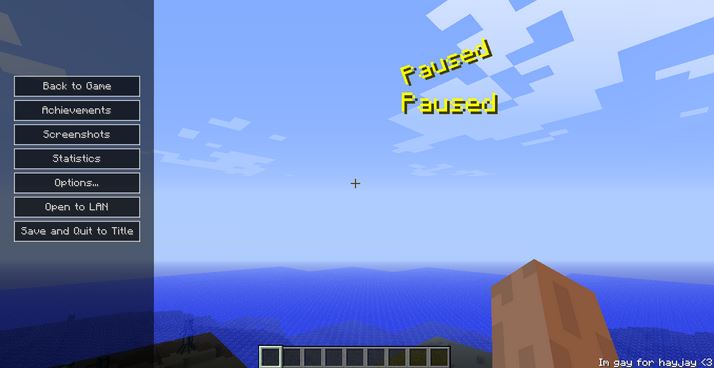This is a finely detailed screenshot from the popular video game "Minecraft." At the center of the image, the game is paused, indicated by the word "Paused" in distinct yellow font. On the left side, a comprehensive options menu is displayed, listing several selections in order: "Back to Game," "Achievements," "Screenshots," "Statistics," "Options," "Open to LAN," and "Save and Quit to Title."

In the bottom right corner, a personal message reads "I'm gay for Hey Jay," adorned with a heart emoji, adding a touch of personalization to the scene. The bottom of the screen shows the character's empty item inventory, a staple visual in Minecraft gameplay.

The view from the character's perspective reveals a scenic vista, likely an ocean, suggesting that the character is positioned on a hill or elevated terrain. You can also see a portion of the character's hand, which is brown in color, consistent with the game's blocky aesthetic. Centrally, a crosshair is visible, standard for aiming and interacting within the game.